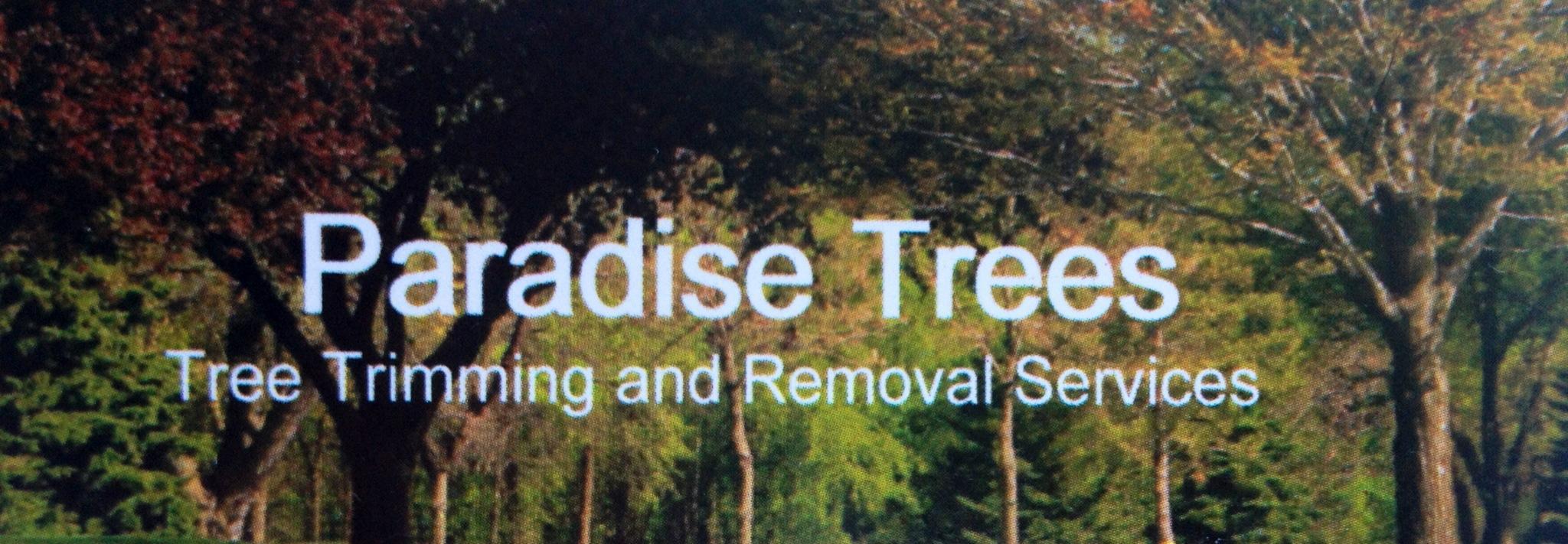The image appears to be a website banner or advertisement for Paradise Trees, a tree trimming and removal service. It features a horizontal, rectangular photograph of various trees as the background. The trees have a diverse range of foliage colors, including green, brown, yellow, and even crimson and burgundy, with visible tree trunks. The picture is somewhat blurry and filtered, giving it a dreamy, soft-focus effect. Superimposed in the center of the image is clean, white sans-serif text. The prominent text reads "Paradise Trees" with a larger font size, while smaller text below states "Tree Trimming and Removal Services." This text takes up approximately a third of the entire image, making it the main focal point. The overall composition suggests that the image could serve as a company advertisement or the header banner on the Paradise Trees website, where visitors might book their services.